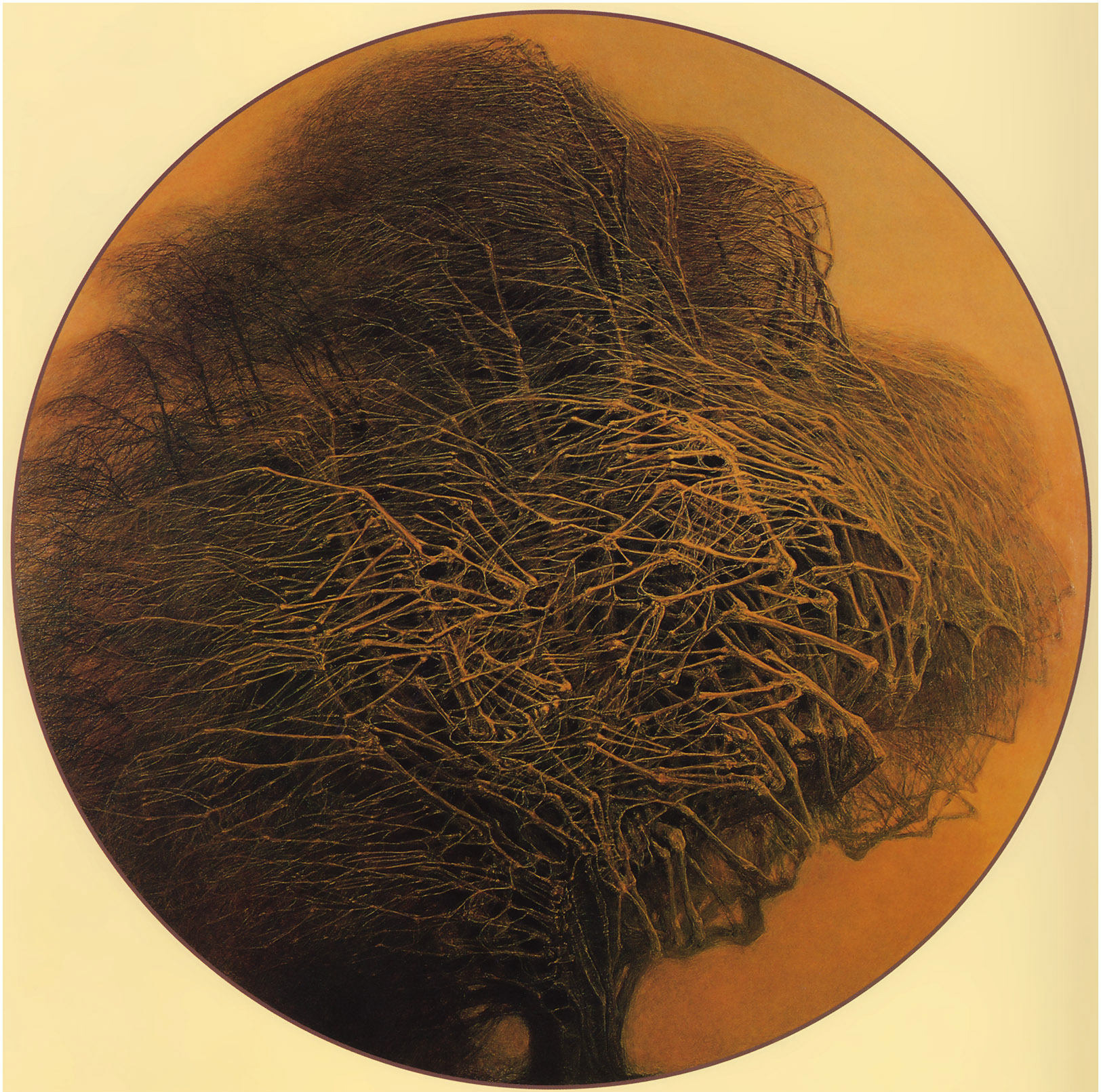The image depicts an abstract and evocative portrayal of a tree during a fierce windstorm. Framed by a solid yellow square background, the central focus is an amber-orange circle that occupies the entire space. Within this circle, a tree rendered in shades of brown and dark hues appears to be caught in a tempest, with its branches and leaves dramatically swept from right to left. The scene is enriched by a deep burnt red tone, giving the sense of a dust storm amidst a blizzard. The tree itself seems almost skeletal, with intricate, crisscrossing twigs resembling bones being tossed by the wind, creating an eerie and surreal appearance. Toward the bottom of the circle, the tree's trunk is partially visible, grounding the chaotic movement above. The image melds realism with abstraction, as the storm-blown branches form an intricate web that requires a closer look to discern the composite shapes of multiple intertwined trees, ultimately coalescing into a single, hauntingly beautiful tree.